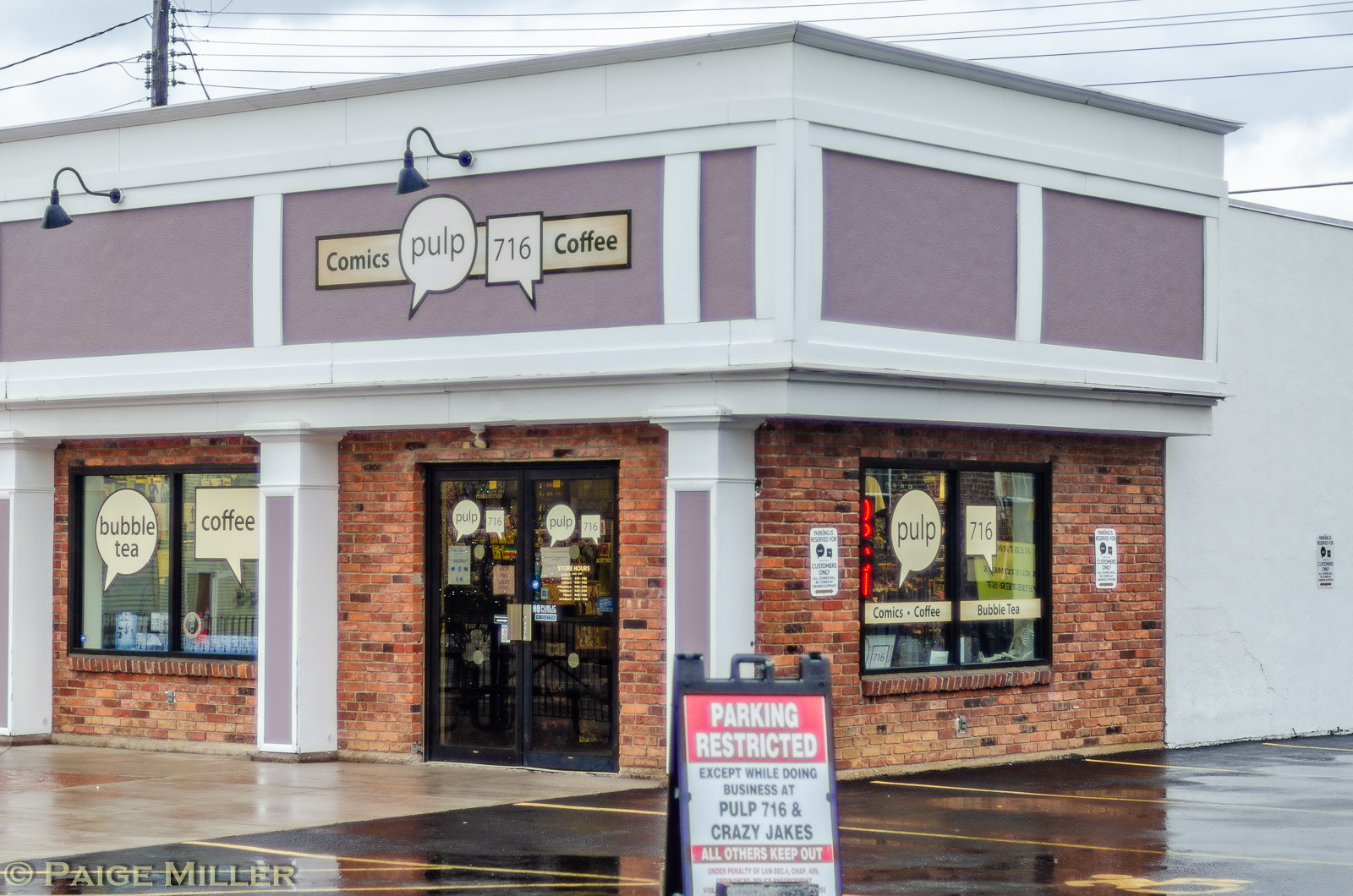The photograph depicts an angled, outdoor view of a comic book and coffee store named "Pulp 716 Comics Coffee" on an overcast, rainy day. The store features a red-orange brick facade with white columns intermittently placed along the walls. Each column is adorned with purple stripes, and above the entrance, there is a signboard with a white background containing purple squares. One prominent square reads "Comix Pulp 716 Coffee." The front of the store is flanked by large clear windows with black door frames, displaying various word bubbles that advertise items like "Bubble Tea," "Coffee," "Pulp," and "716." In the wet parking lot covered with black asphalt and marked by yellow lines, a black plastic warning sign stands out. It reads "Parking Restricted" at the top in white text, followed by "Except While Doing Business at Pulp 716 and Crazy Jake's," with a final cautionary note stating "All Others Keep Out." Telephone poles and wires span above the building, accentuating the gloomy, cloud-filled sky. Despite the wet conditions, the vivid details of the store's exterior signage and layout are clearly visible.